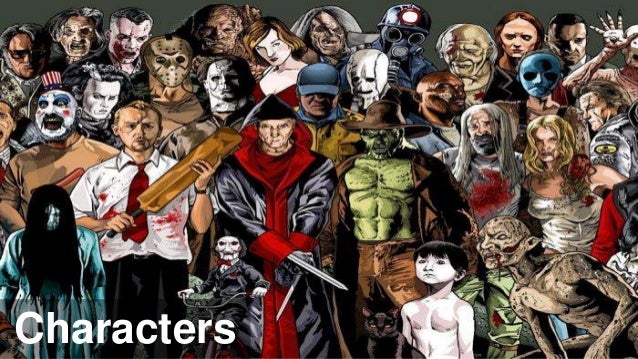This highly detailed graphic illustration conveys a chaotic and macabre scene filled with a variety of characters that appear to be from a mix of comic books, movies, or video games. These characters, spread across four rows, showcase a nightmarish tableau that features approximately eight to ten figures per row, with about four in the frontmost row. A prominent element in the lower-left corner is the white text "characters," succinctly labeling the depicted ensemble.

At the center of this imagery, a black cat catches the eye, while surrounding it, one can see distinct characters: a man grievously wounded in the chest on the right, a bloody woman, individuals in ski masks, and demon-like figures, including a goblin to the left and a green goblin in the center. There’s even a sinister cowboy and a man wielding swords. On the left side, there’s a terrifying figure, dressed in a suit and tie, holding a bat and covered in blood. Another eerie presence is a lady with hair obscuring her face, and nearby, a grotesque clown. Emphasizing the multifaceted terror, a figure with a gas mask looms at the top, while a psychopath appears alongside a forlorn, shirtless boy gazing upwards. Additionally, a ghoul can be seen riding a small bicycle, further adding to the surreal horror.

The characters, filling the entire frame, represent a blend of human and monstrous entities, all depicted with graphic intensity, making it clear that the scene is one of extreme chaos and horror. The meticulous artwork captures the unsettling essence of a world overtaken by blood, violence, and otherworldly figures, rendering a vivid and disturbing visual experience.